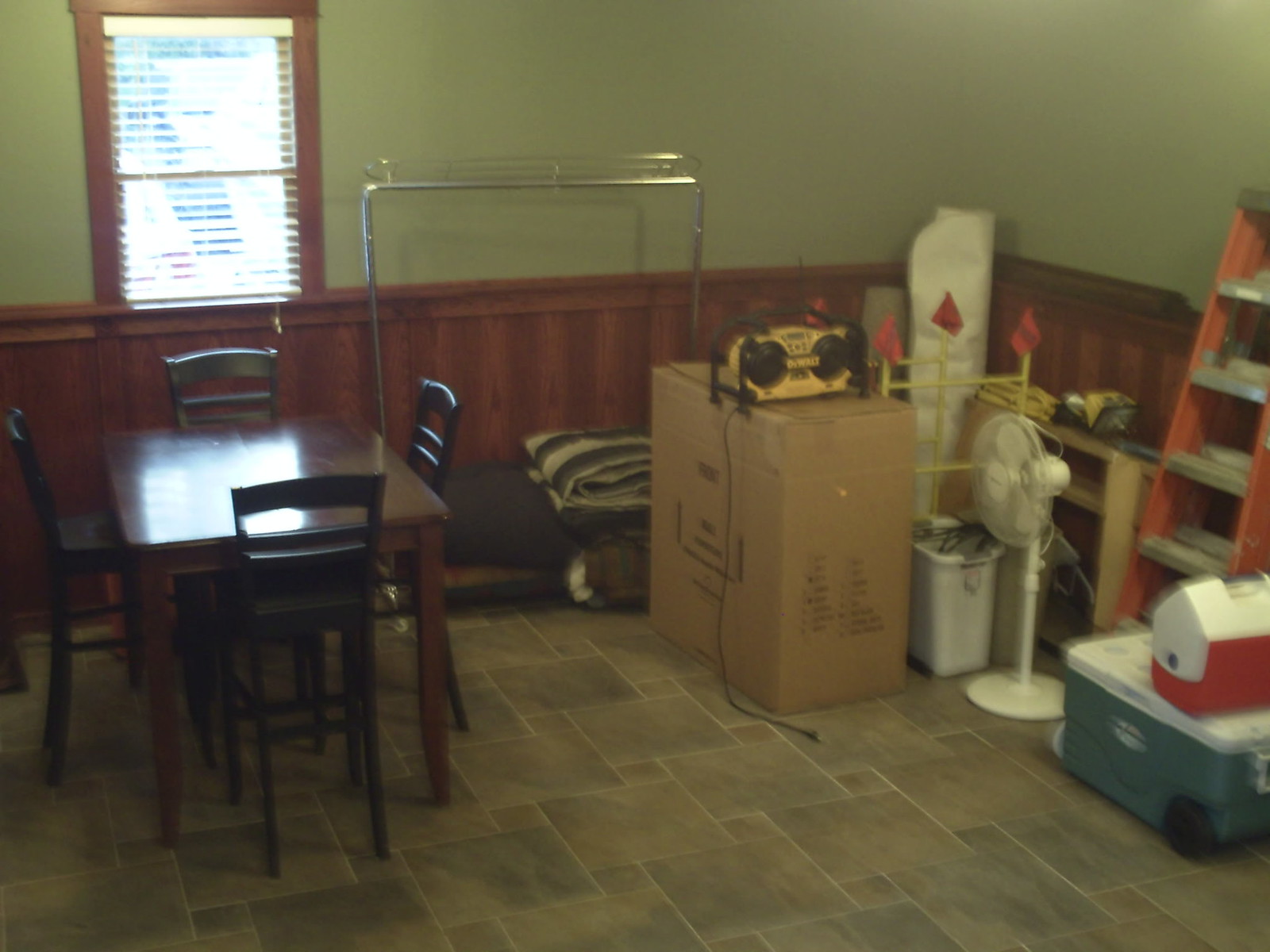The rectangular photograph, oriented with its longer side running left to right, captures the interior of a room characterized by greenish walls adorned with brown wood wainscoting that rises to about waist height, topped by a chair rail. The window on the left side of the image is framed in wood, and the blinds within it are open, allowing a substantial amount of light to flood the room. The floor is covered in a pattern of gray and brown tiles.

On the left side of the room stands a dining table accompanied by four chairs, with a reflective surface that gleams. A window allows natural light to spill over this setup. Centrally located on the back wall is a rack designed to hold clothing, currently supporting a blanket at its bottom. Below this rack, a closed cardboard box occupies space, and a yellow DeWalt radio rests on top of it.

Moving towards the right side of the room, a stand-up fan and a small waste paper basket filled with what appears to be cords come into view. Nearby, a yellow framing structure adorned with red flags catches the eye. Additionally, a roll of plastic wrap lies in the background alongside a small shelf. The bottom right of the image reveals a couple of coolers and a ladder leaning against the right-hand wall.